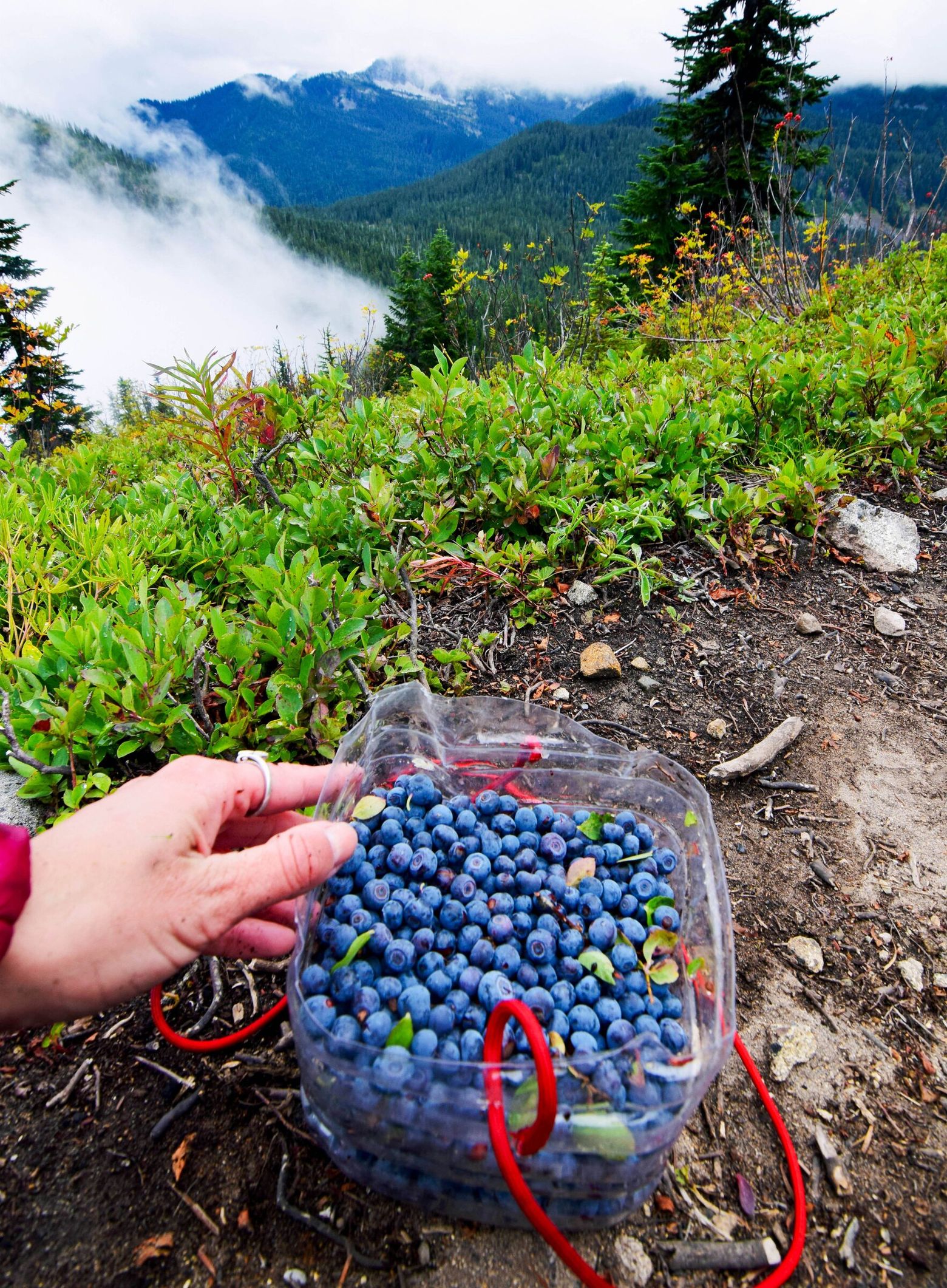In this photo, a nearly full, clear plastic bucket brimming with small, wild blueberries rests on the forest floor. The container, equipped with two red straps, features a scattering of leaves and twigs among the berries, adding a touch of authenticity to the harvest. A Caucasian person's left hand is gently touching the bucket, suggesting they spent a considerable time picking these berries in the wilderness. The background reveals a scenic, mountainous landscape with a forested trail and numerous trees. Misty valleys and clouds hover over the mountain tops, indicating a high elevation and a somewhat cloudy day. The scene hints at a tranquil, forested environment ideal for hiking and berry picking.